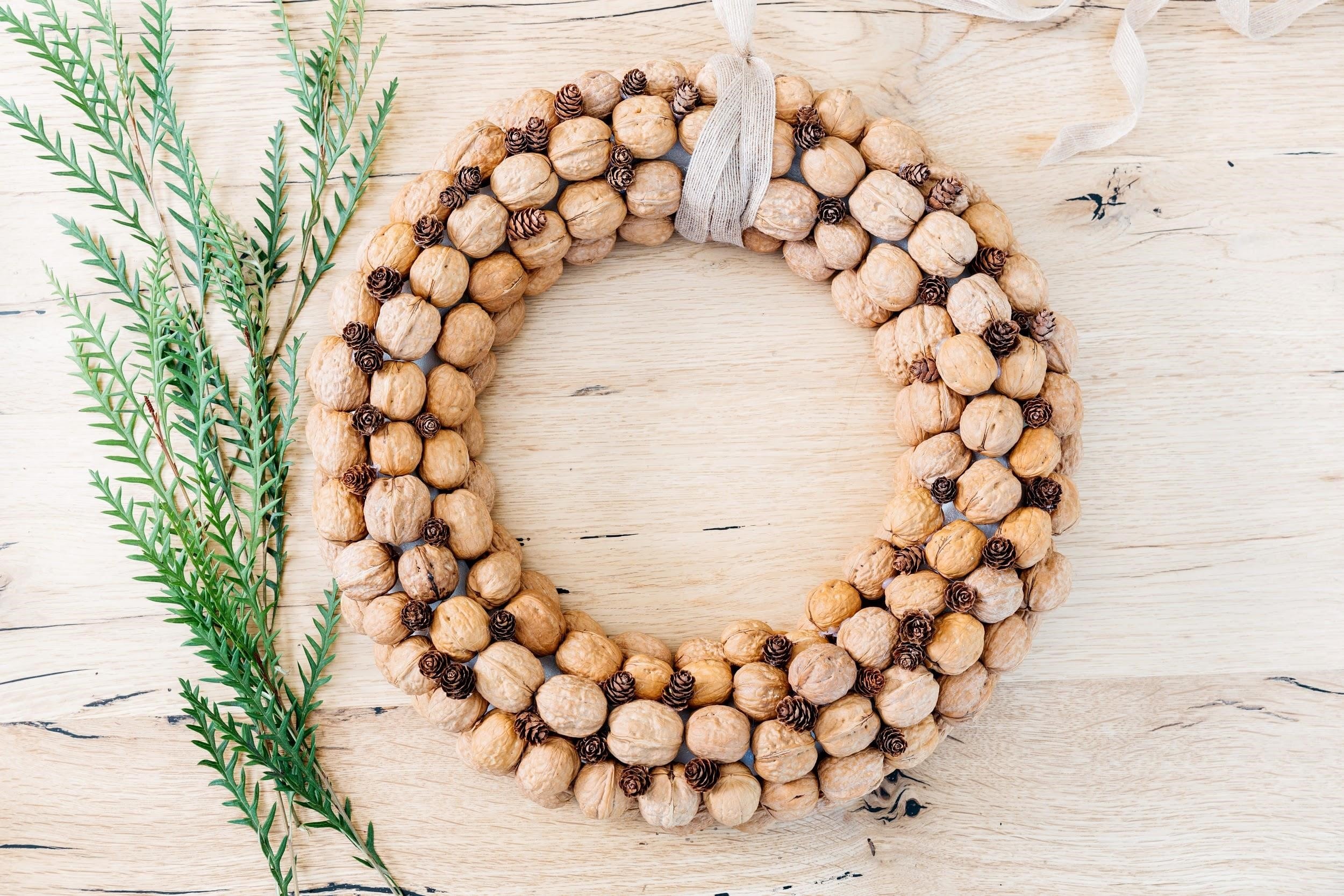In this detailed product photo, we see a circular headwear-like decoration crafted from an assortment of beads, tiny acorns, and walnuts, forming three to four concentric circles. These brown beads and nuts are intricately interwoven, creating a transparent effect in places. The top part of the wreath features a piece of net-like fabric, or possibly a thin, flat rope, that ties everything together. Lying beside the wreath on the left, we see a plant with thin, green leaves resembling spikes, adding a delicate contrast. All these items are placed on a light brown, natural wooden tabletop, marked with cracks and indentations, enhancing the rustic aesthetic.